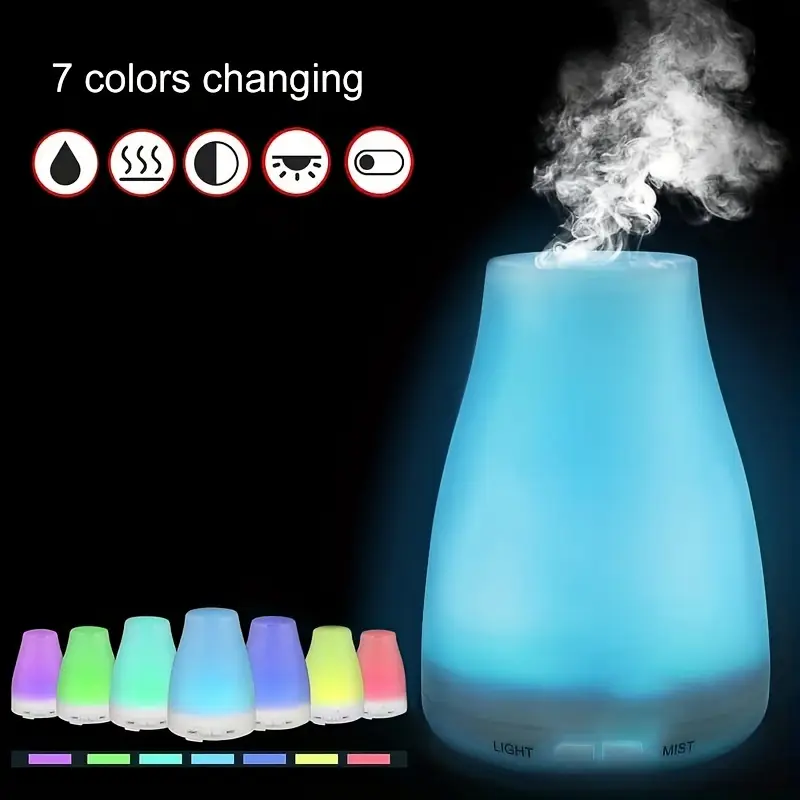The advertisement poster showcases a sleek, blue oil diffuser prominently positioned on the right side against a black background. This diffuser, resembling a bottle, emits a delicate stream of white smoke from its narrow top. The base of the device is wider, featuring two buttons labeled "light" and "mist." On the left side of the image, there is a lineup of seven additional diffusers in an array of vibrant colors, including purple, green, blue, yellow, red, cyan, and lavender. Below these diffusers, a color scale further highlights the range of available hues. In the top left corner, white text declares "7 Colors Changing," accompanied by five circular icons representing various features like a water droplet and brightness. This visually striking composition, with its array of colorful diffusers and clear functional labels, effectively communicates the product's aesthetic and multi-color lighting options.